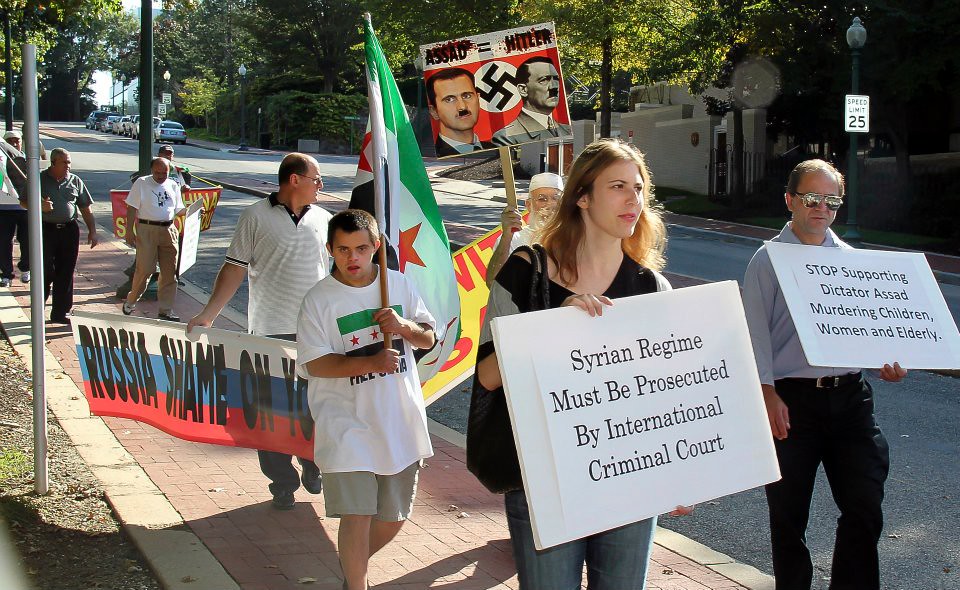The photograph captures a vivid and dynamic scene of people protesting on a brick-paved sidewalk that begins at the top left and extends to the bottom right corner of the image. The sidewalk features reddish-brown bricks bordered by gray ones. To the right of the sidewalk, a road with two lanes is separated by an elevated red brick barrier.

At the forefront of the protest are a woman with dark blonde, wavy hair wearing a black shirt, and a man wearing sunglasses. Both are holding large white rectangular signs with black print. The woman’s sign reads, "Syrian regime must be prosecuted by International Criminal Court." The man's sign states, "Stop supporting dictator Assad murdering children, women, and elderly." Directly behind them, a young boy in a white shirt holds a flag with green, white, and black stripes and red stars. 

Adjacent to the boy, a protester displays a provocative sign featuring photos of Assad and Hitler, separated by a Nazi symbol, with red paint resembling blood splattered across it. The sign reads "Assad = Hitler," implicating Assad with historical atrocities.

Further back in the group, another man carries a wide banner with the inscription "Russia shame on you" in black letters, emblazoned across white, blue, and red stripes. The line of protesters continues behind him, holding various signs and banners, creating a sense of solidarity and urgency. The protest occurs on a sunny day, with trees, bushes, and a few buildings lining the street, and cars parked along the roadside.